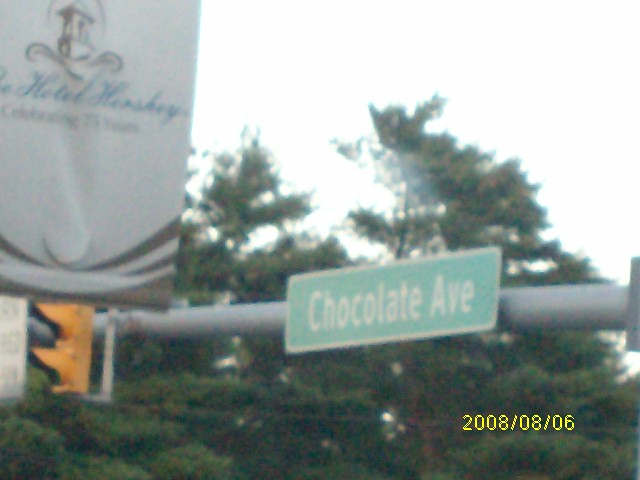The image prominently features a road sign hanging off a horizontal gray pole that also supports a traffic light. In the bottom right-hand corner, the date "2008/08/06" is displayed in yellow text. The gray pole extends horizontally from the right, where a rectangular road sign with a very light green background reads "Chocolate Ave" in white lettering. To the left of this sign is the bottom portion of a yellow traffic sign. Above this, in the top left, is a white sign with brown stripes at the bottom, adorned with indiscernible blue cursive writing. The background showcases dark green trees and a white sky.